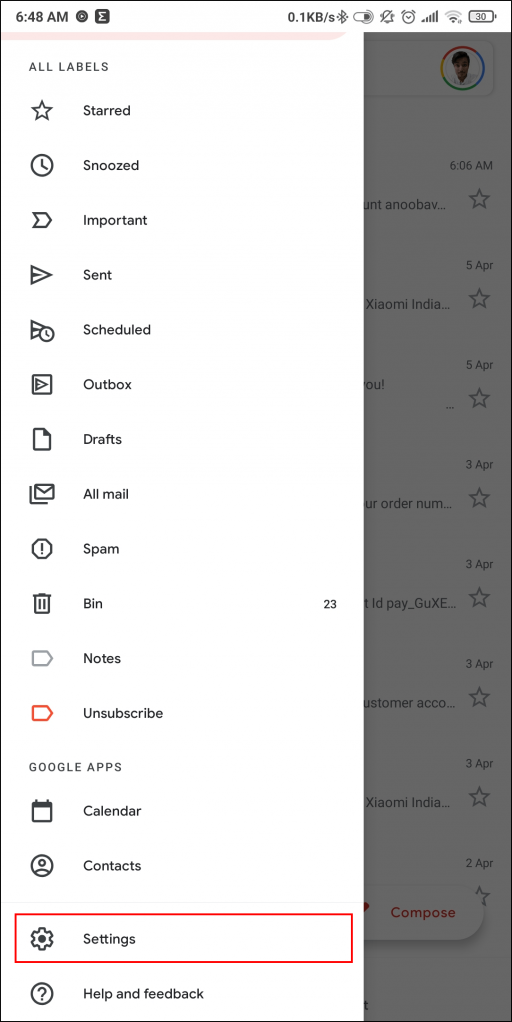This digital image depicts a screenshot taken at 6:48 AM, with the device’s battery level at 30% and a Wi-Fi connection showing full bars. At the top of the screen, the "All Labels" section is highlighted. Below that, a series of labels and their corresponding icons are shown, including:

- Starred (indicated by a small star icon)
- Snoozed (represented by an alarm clock icon)
- Important
- Sent
- Scheduled
- Outbox
- Drafts (accompanied by a piece of paper icon)
- All Mail (represented by an envelope icon)
- Spam
- Bin (displaying a trash can icon) with a count of 23 items
- Notes
- Unsubscribe

Additionally, there is a section for Google Apps which includes:
- Calendar (represented by a tiny calendar icon)
- Contacts
- Settings (outlined in red)
- A Help and Feedback option marked with a question mark icon